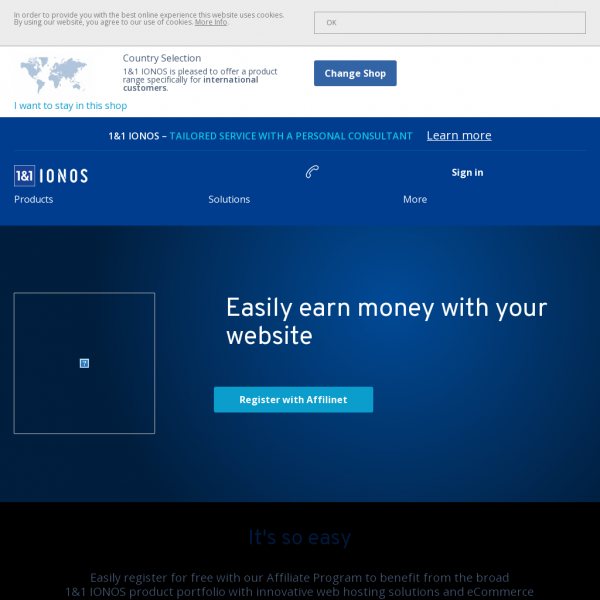The image is a screenshot of a webpage, featuring a notification bar at the top with a gray background. The notification reads: "In order to provide you with the best online experience, this website uses cookies. By using our website, you agree to our use of cookies. More info." A small input box labeled "OK" is also present.

Below the notification, a white bar on the left-hand side displays a gray map of countries and a section labeled "Country Selection." It states, "IONOS is pleased to offer a product range specifically for international customers," accompanied by a blue button that says "Change shop" and a link that says "I want to stay in this shop."

The main section of the page features a bluish background. At the top, it states: "1&1 IONOS tailored service with a personal consultant," with an option to "Learn more." The 1&1 IONOS logo, consisting of "1&1" in a square and "IONOS" in white capital bold letters, is situated on the left.

A navigation menu with options such as "Product," "Solutions," "More," and "Sign-in" is seen. Under this, there is text promoting affiliate marketing: "Easily earn money with your website," followed by a blue button that says "Register with Affiliate Net" in white text.

On the left-hand side, there is a gray-bordered box where the image hasn't loaded, accompanied by the text "It's so easy" in blue at the bottom.